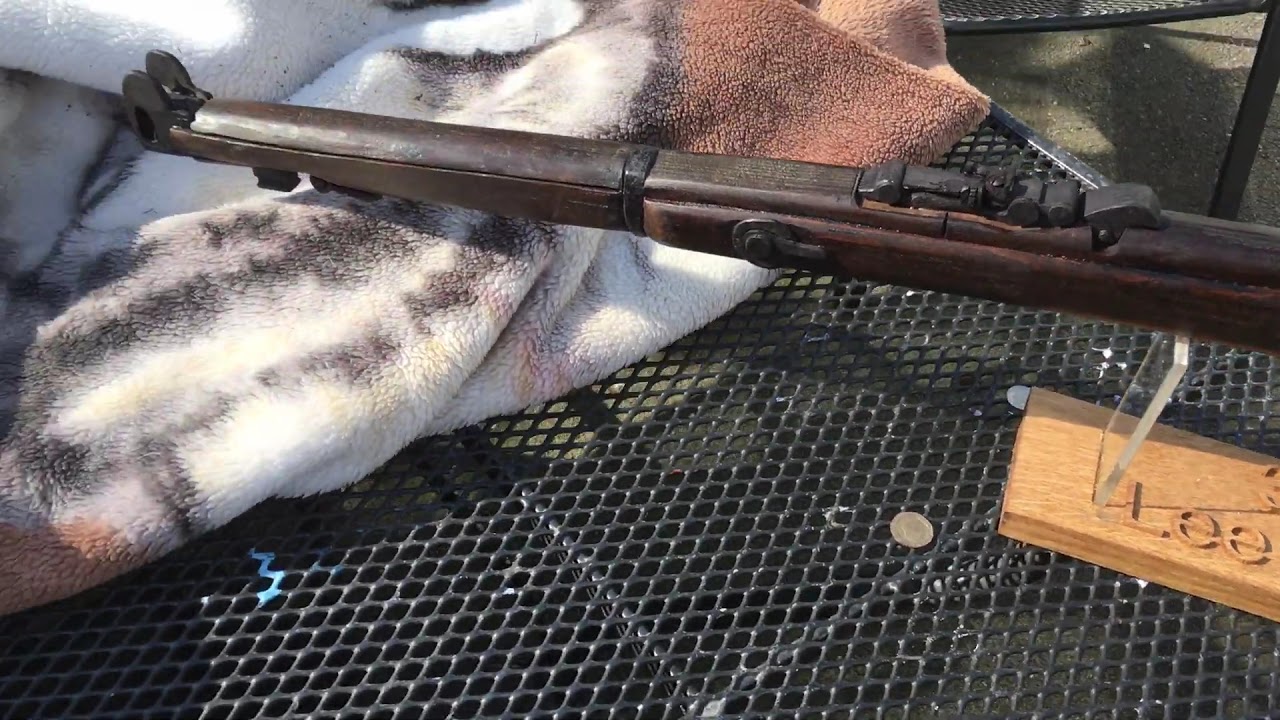In this image, there is an old rifle prominently displayed, pointing towards the upper left. The rifle, consisting of wooden and metal parts, appears worn with a visible seam or crack on the barrel, indicating its age. The rifle is partially propped up by a wooden block with a plexiglass section, and the block has the letters "L.E.E." engraved on it. The rifle rests on a colorful, soft blanket with a brown, white, and black pattern, which is draped over a metal wire table. This table, with its grid-like structure, allows visibility to the ground below. Also present on the table are a few coins, including what looks like a quarter and another smaller coin, possibly a nickel or a dime. The scene is illuminated by sunlight, casting distinct shadows of the objects onto the table.